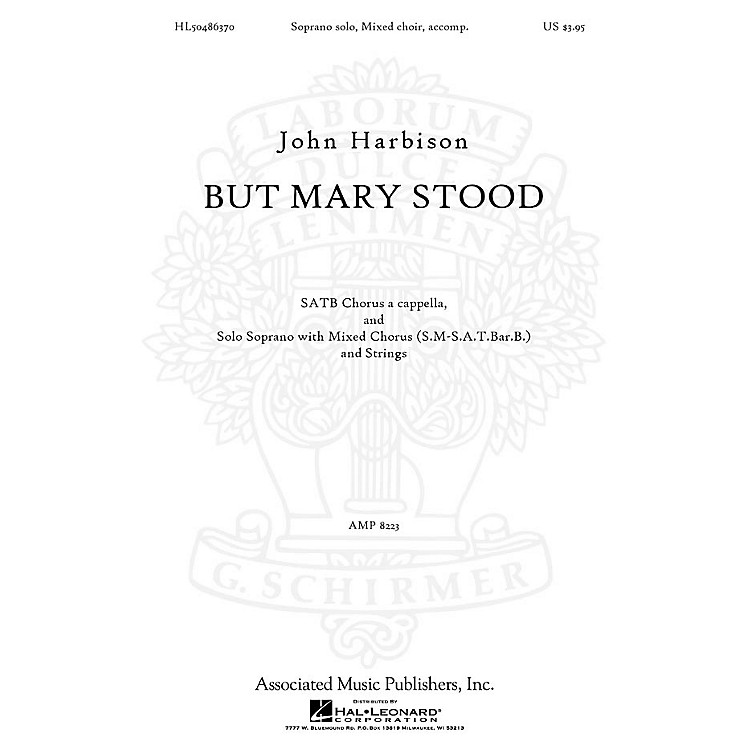This image depicts the cover page of a piece of choral sheet music. The background is predominantly white, with various lines of black text providing essential information about the composition. In the top left corner, the catalog number "HL50486370" is displayed, while the top right corner indicates the price as "US $3.95." 

Centralized text prominently features the composer's name, "John Harbison," followed by the title "But Mary Stood" in all capital letters. This is the most noticeable text on the cover, drawing immediate attention. Below this, in smaller black text, the musical arrangement is detailed: "SATB Chorus A Cappella and Solo Soprano with Mixed Chorus (SM-SATB) and Strings." Further down, the AMP number "8223" is noted.

At the bottom, the publishers are listed as "Associated Music Publishers, Inc." and "Hal Leonard Corporation," alongside their respective logos. There's also a faint, grey background image featuring a harp surrounded by floral elements and a banner with the inscription "Laborum Dulce Lenumen." The publisher's name "G. SCHIRMER" is also visible in a banner at the bottom of this background image.